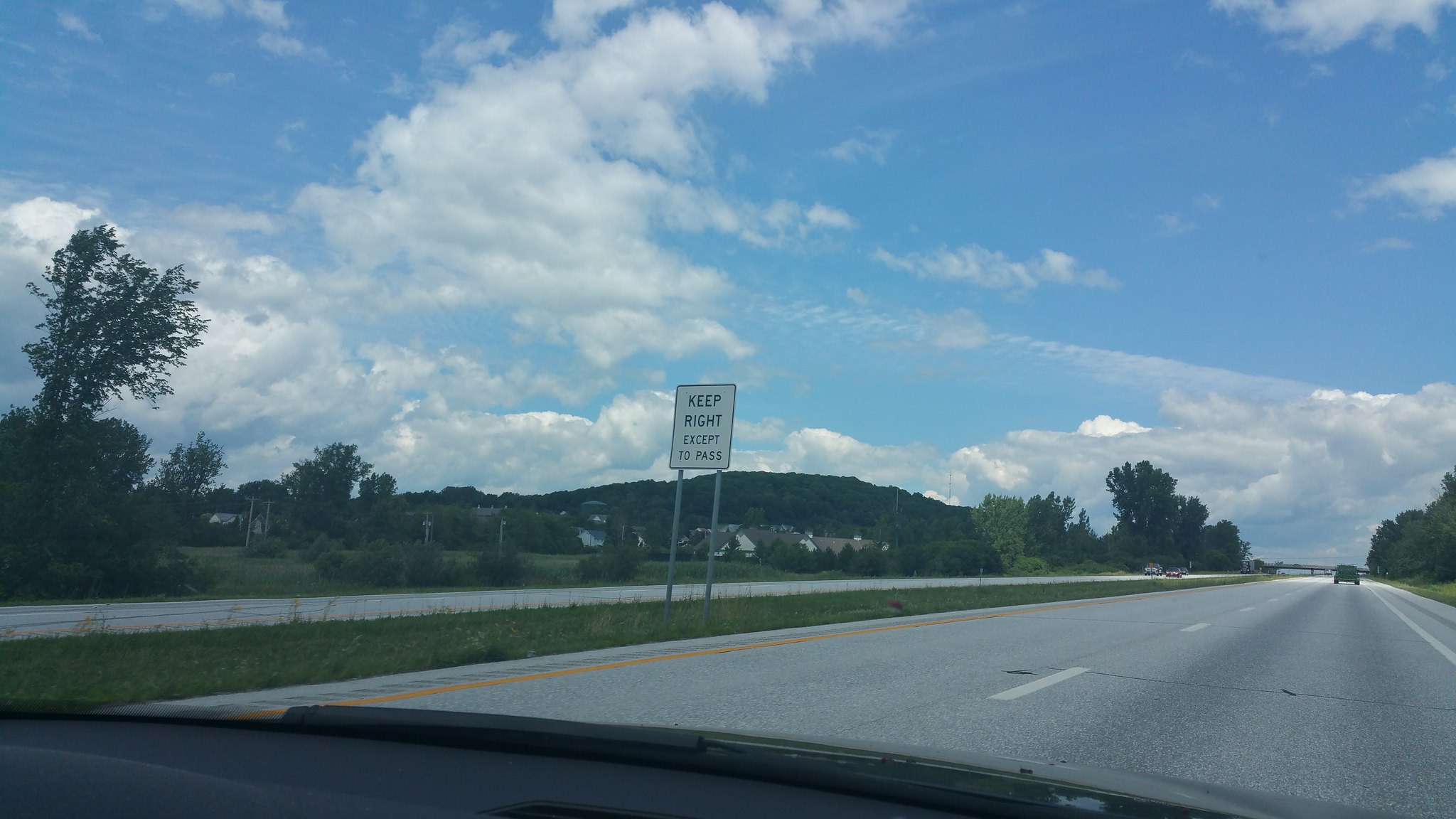The image captures a detailed view of a roadway as seen from inside a passenger vehicle, presumably taken from the right side of the vehicle. The vehicle is traveling down the right lane of a divided highway, which features two lanes in each direction. 

In the foreground, we can glimpse the dark-colored dashboard and a portion of the windshield wiper, indicating the camera's interior position. The camera is aimed towards the center of the road, where a white road sign reads "Keep Right Except to Pass" in black lettering. 

The highway appears to be flanked by a mix of trees and grassy areas, contributing to a scenic yet somewhat rural atmosphere. On the oncoming lanes, several vehicles can be seen in the distance, though their specifics are indiscernible due to the distance. In the lane the camera-equipped vehicle is traveling, there is a car ahead but too far away for detailed observation.

The right side of the highway is bordered by a solid white line, while the center lane is demarcated by a broken white line. To the left, hints of a small residential community are visible, with light-colored houses partially obscured by foliage. A tall hill rises in the distance, adding a measure of elevation to the otherwise flat terrain. 

The weather is bright and sunny, yet scattered with patches of white and gray clouds, painting a partly cloudy sky above the traveling vehicle.